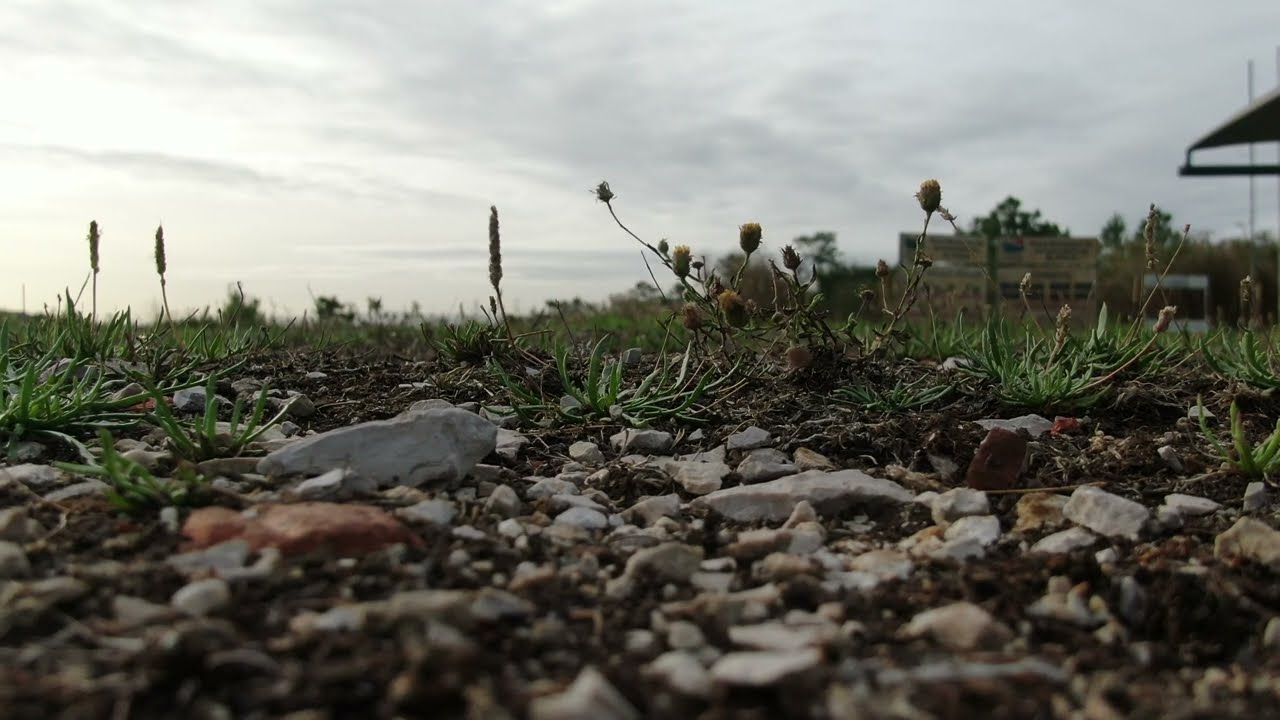The image is captured from a ground-level perspective, with the camera seemingly placed among the pebbles and gravel. The foreground is dominated by a variety of rocks, showcasing diverse shapes and colors, including white, gray, brown, maroon, and tan. Scattered among the stones are three sprigs of weeds, jutting out just left of the center, with some small flowers beginning to emerge. The background reveals a grassy area, hinting at some greenery despite the rocky terrain. Far in the distance, there appears to be a blurred sign or billboard, difficult to discern in detail. Overhead, the sky is overcast, blanketed by gray clouds. The overall scene portrays an outdoor setting, blending earthy textures with subtle hints of life amidst a rocky, partially grassy landscape.